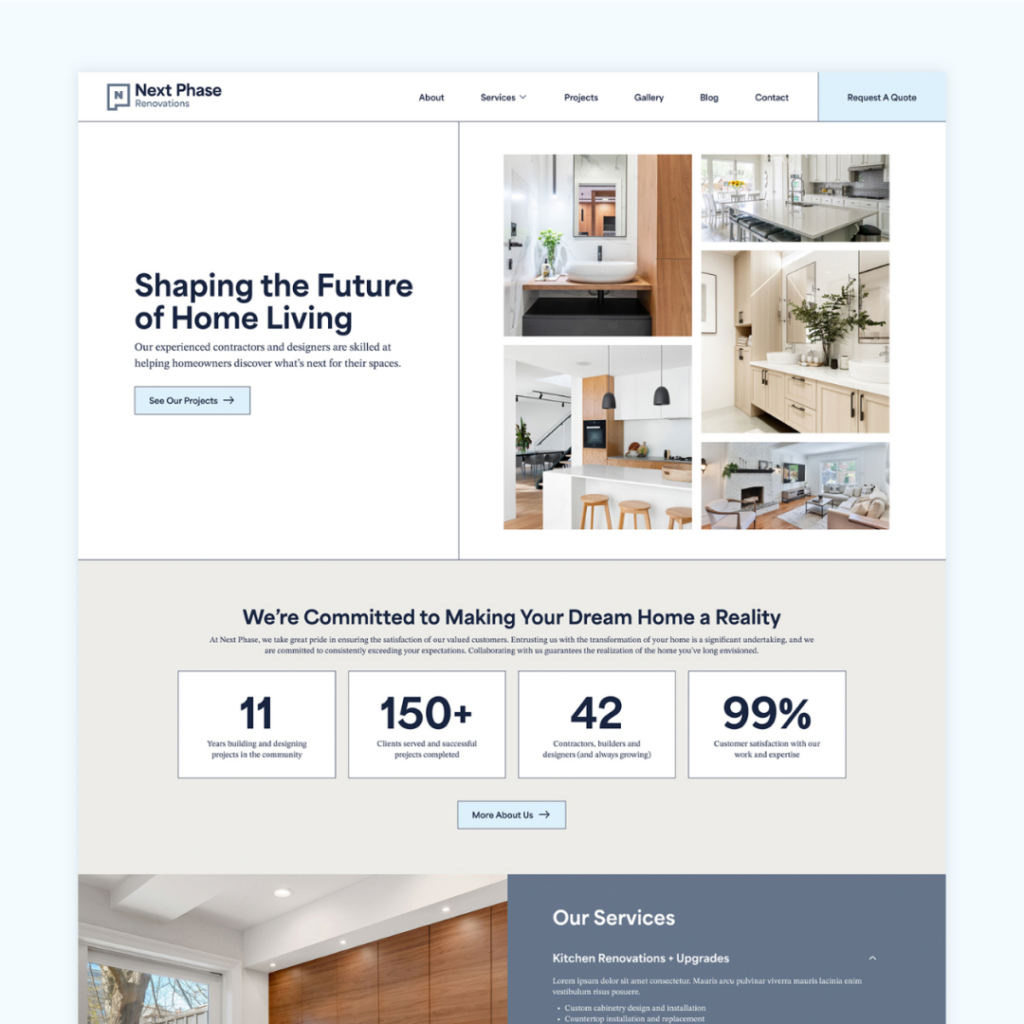This is a detailed caption for an image of a webpage for Next Phase Restorations:

---

The screenshot features a webpage encased in a light blue border, with a predominantly white and beige background. In the top left corner, the company name "Next Phase Restorations" is prominently displayed. Adjacent to this, a navigation menu lists options: About, Services, Projects, Gallery, Blog, and Contact. On the top right, there's a "Request a Quote" button. 

Centered on the page, a text box reads: "Shaping the Future of Home Living. Our experienced contractors and designers are skilled at helping homeowners discover what's next for their spaces." Beneath this text, a button labeled "See Our Projects" is accompanied by a right arrow icon.

To the right of this text box, a collage of five images showcases different rooms. The arrangement includes two square images on the left side, two smaller rectangular images—one at the top and one at the bottom—and another square image in the center. These images depict various interiors, including bathrooms, kitchens, and living rooms.

Positioned below this content, against a beige section of the background, is the statement: "We're committed to making your dream home a reality," followed by some small, barely legible subtext. There are four boxes with numbers: "11," "150+," "42," and "99," each accompanied by its own subheading. Another button labeled "More About Us," also with a right arrow icon, is located below these boxes.

Finally, at the bottom of the webpage, partially cut off by the frame, there is text on the right side detailing "Our Services: Kitchen Restorations and Upgrades," alongside an unspecified image to the left. The additional information here is not readable.